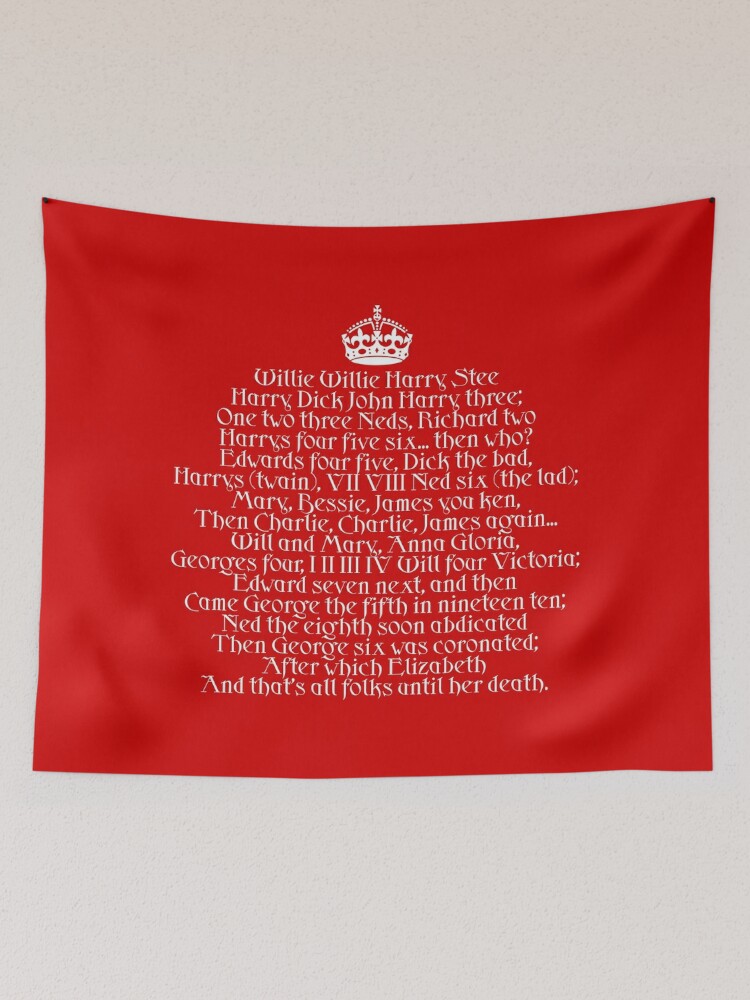This is an image of a bright red, slightly rectangular cloth banner hanging against a white wall. The banner, which appears to be secured in the upper left and right corners with dark pushpins, prominently features a white crown symbol centered at the top. Below the crown, there is detailed, white textual content in a slightly fancy font, listing names and numbers, most likely representing a historical or mnemonic sequence of British monarchs. The text includes: "Willie, Willie, Harry, Steve, Henry, Dick, John, Harry, 3, 1, 2, 3, Neds, Richard, 2, Harrys, 4, 5, 6, then Who, Edwards, 4, 5, Dick the Bad, Harrys Twain, 7, 8, Ned 6 the Lad, Mary, Bessie, James, you can, Charlie, Charlie, James again, Will and Mary, Anna, Gloria, George 4, 1, 2, 3, 4, Will 4, Victoria, Edward 7, next and then George V in 1910, Ned VIII soon abdicated, then George VI was coronated, after which Elizabeth," finishing with the note, "and that's all folks until her death." The overall presentation of the banner gives a historic and scholarly impression.